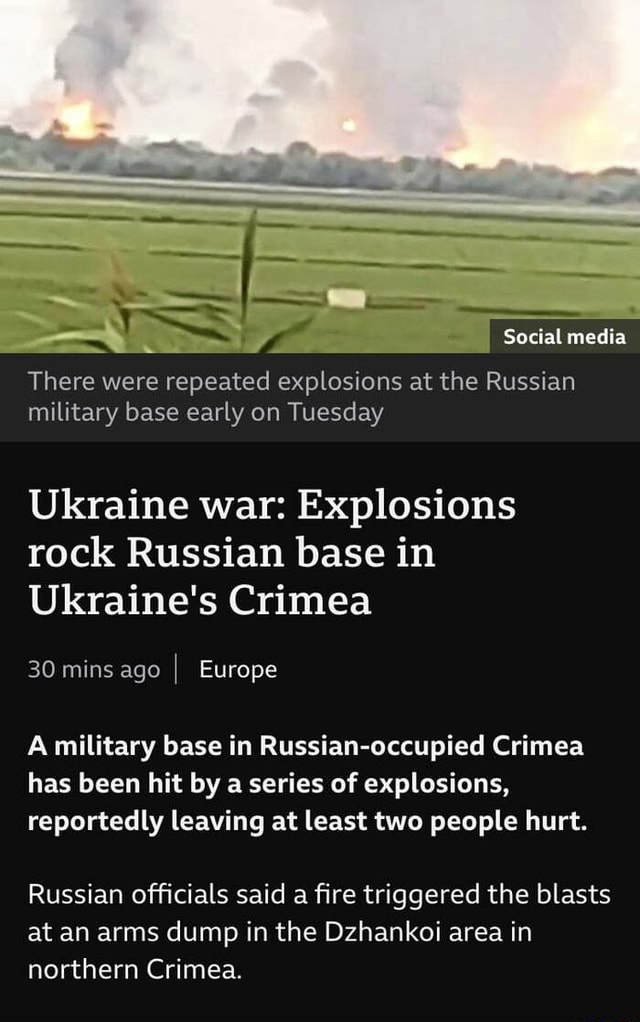Caption: 

A screenshot from a tablet or desktop displays a news article headlined "Ukraine War: Explosions Rock Russian Base in Ukraine's Crimea." The image portrays a field with blurry green plants in the foreground and trees in the background, with visible smoke and flames indicating a fiery incident. The article, tagged under social media and Europe, reports on repeated explosions at a Russian military base in the Zakhnoye (Dzhankoi) area of northern Crimea. According to Russian officials, a fire at an arms dump triggered the blasts, resulting in at least two injuries. The news was published thirty minutes ago, with varying boldness in the white text emphasizing different parts of the report.